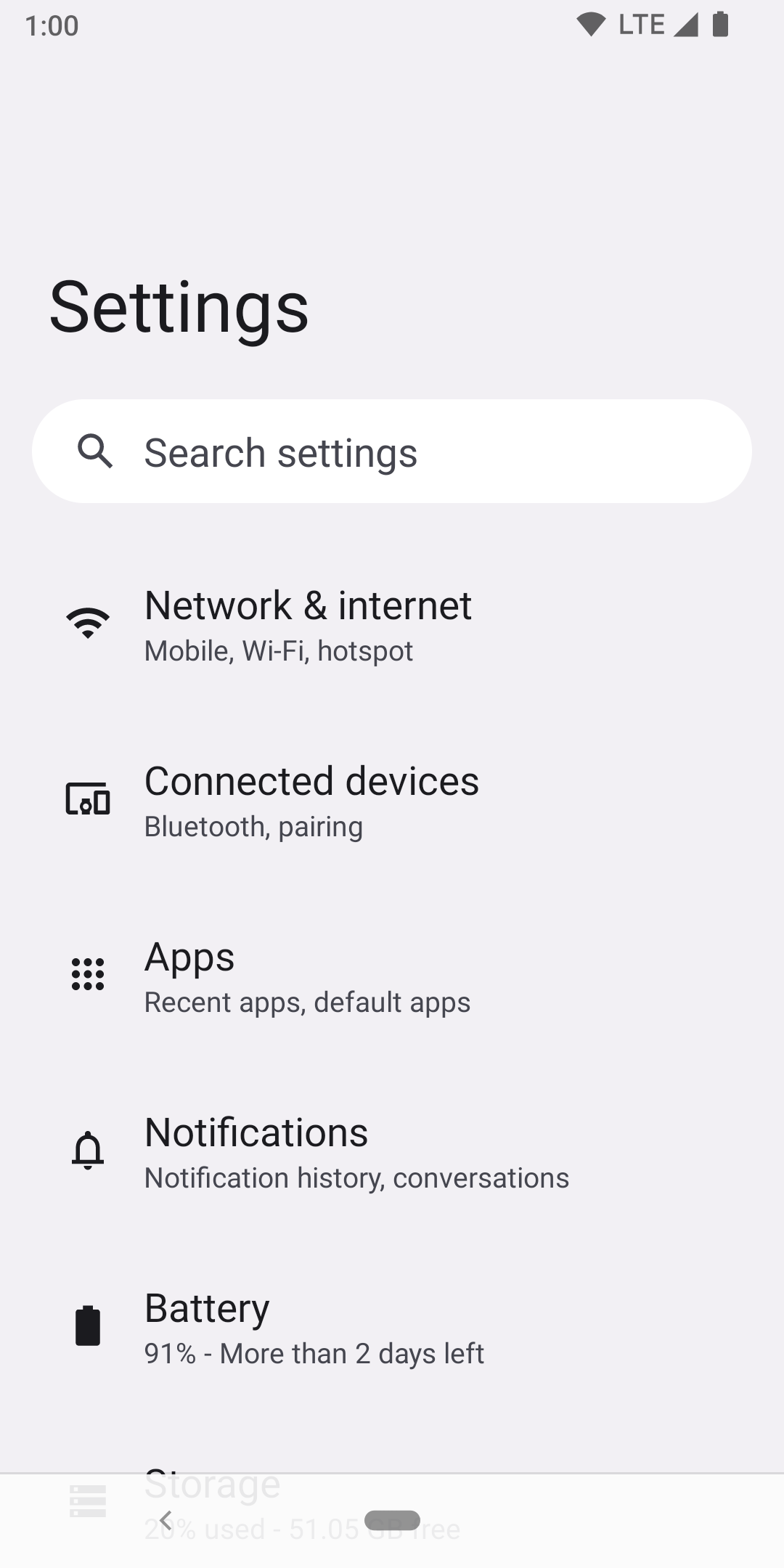Screenshot of a Mobile Device Interface at 1:00 PM with Detailed Settings Display

The image captures a screenshot from a mobile device, specifically showcasing the time as 1:00 PM, displayed in the upper left corner. Adjacent to the time on the right side are the LTE signal indicator, Wi-Fi icon, and battery icon, which reads 91%, suggesting more than two days of battery life remaining.

The background of the screen is a very soft, pastel shade that leans towards light lilac or pink. Prominently displayed in black text at the top is the word "Settings". Immediately below, there is an elongated search box with smoothly curved edges.

The settings menu list includes the following items:
1. Network & Internet
2. Mobile, Wi-Fi, Hotspots
3. Connected Devices
4. Bluetooth Pairing
5. Apps
   - Recent Apps
   - Default Apps
6. Notifications
   - Notification History
   - Conversations
7. Battery, displaying 91% with a note stating "more than two days left".

Each menu item is clearly delineated, making navigation straightforward and indicative of a well-organized user interface.